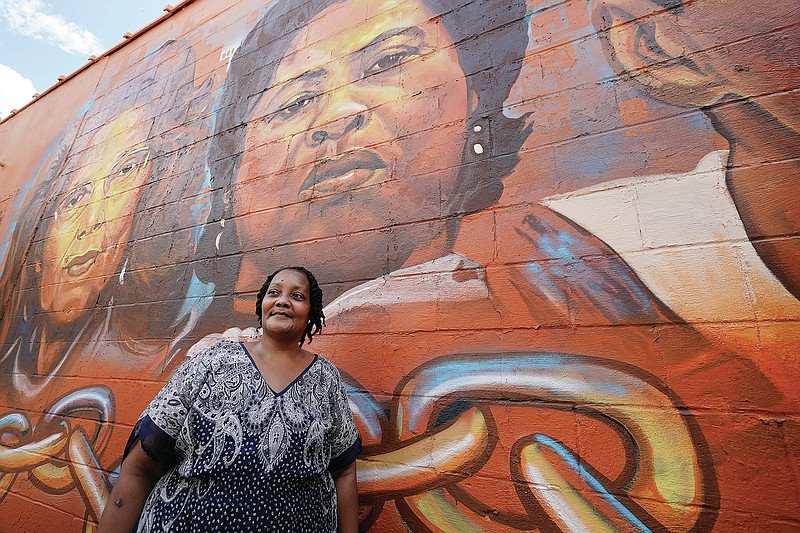In the image, an African American woman stands in front of a detailed brick wall mural in an urban setting. She has short black hair, wears a white and black polka-dotted shirt with dark blue outlines, and has a pleasant smile as she looks to her left. The mural behind her, spanning the entire horizontally rectangular brick wall, features three African American figures predominantly painted in dark browns and rust colors with subtle blue highlights. To her left on the mural, the detailed portrait of a woman with shoulder-length straight hair and clear glasses is depicted with a serious expression and intense stare. Adjacent to her, above the woman's head in the image, is another woman with short black hair. To the right side of the mural, a partially visible figure wears a white shirt, whose gender is indeterminate due to being cut off. The lower portion of the mural illustrates chain links, implying a historical context of enslavement. The mural even incorporates some white bricks on its right side, adding contrast to the overall brown and red hues of the painted brick wall.